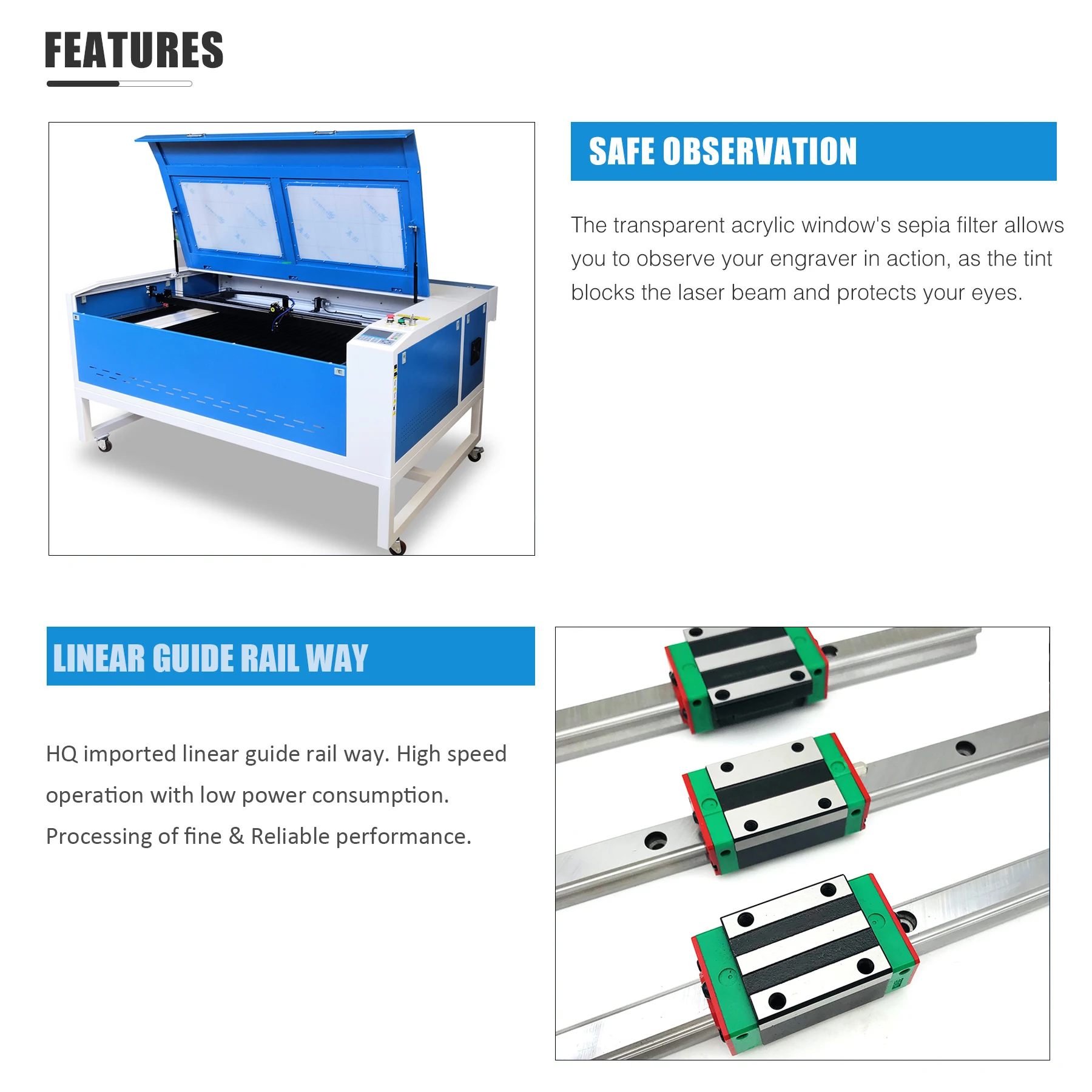The advertisement showcases an HQ imported Linear Guide Railway, highlighting its high-speed operation with low power consumption and reliable performance. Prominently featured is a durable, heavy-duty blue and silver chassis on casters with a hinged lid, resembling a large toolbox with an integrated control panel. Adjacent to this image, in a blue section with white lettering, the ad emphasizes "Safe Observation," explaining that the transparent acrylic window with a sepia filter allows users to safely observe the engraver in action, as the tint blocks the laser beam to protect their eyes. Below this, the ad depicts how the Linear Guide Railway would look when laid out on the floor, showing three silver rails with black, green, and red square attachments, providing a clear illustration of the product's design and functionality. The entire layout is presented against a white background with black text describing its features.